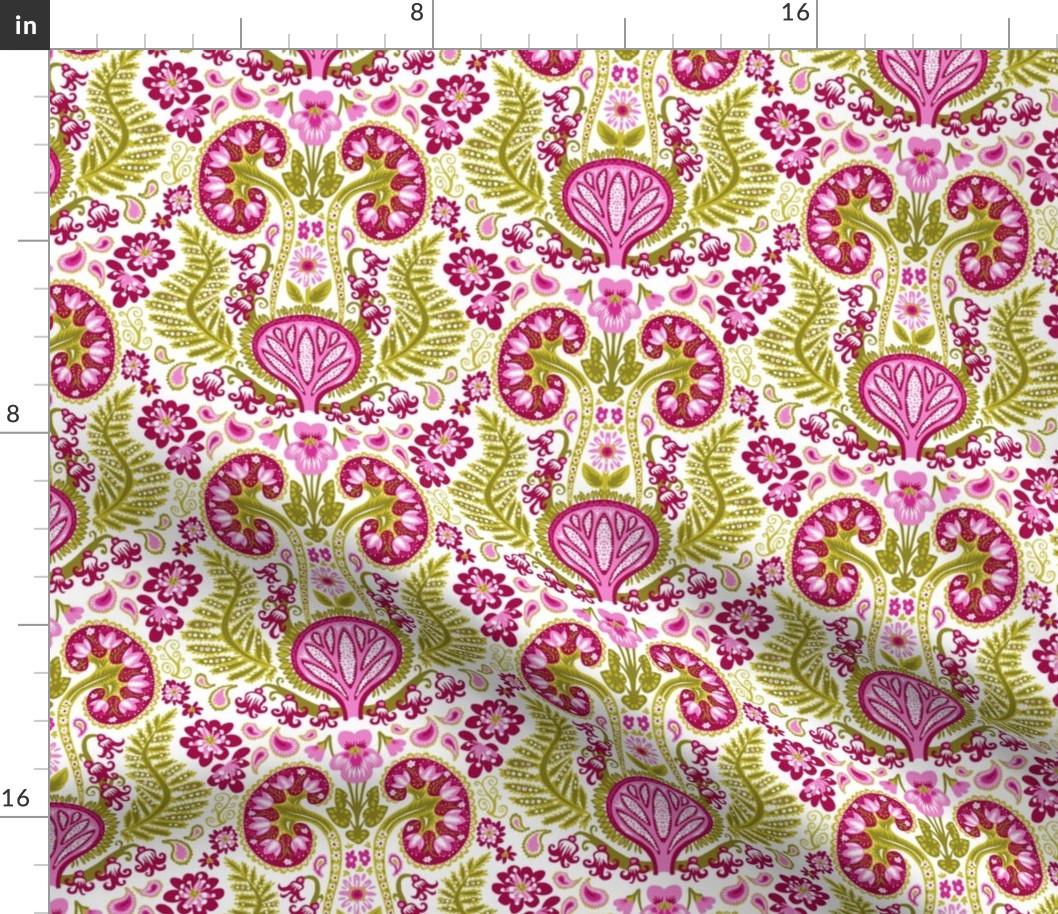The image features a 20x20 inch square piece of fabric with a black border marked in inches, with labels at 8, 16, and additional segments articulating its dimensions. The design is primarily floral, showcasing a vibrant array of colors including magenta, pink, purple, and olive green against a white background. The fabric pattern includes large green leaves and flowers interspersed with purple semi-spirals resembling kidneys and a uterus at the center. These details are surrounded by smaller, intricate flowers and plants that wind from the lower left corner to the top, creating an intricate and continuous design. The fabric appears slightly folded and wavy, not fully flat, enhancing the dynamic nature of the floral and anatomical motifs.